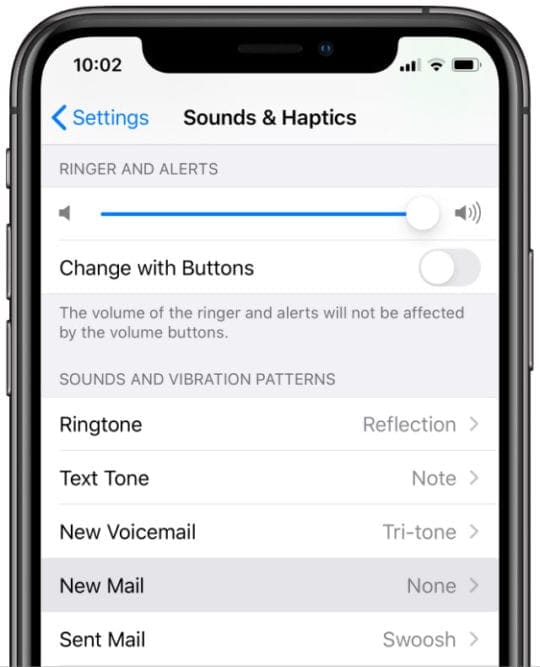This image captures a screenshot of a smartphone screen displaying the "Sounds & Haptics" settings. It begins with a partial view of the phone's interface, where the following details can be seen:

1. **Upper Left Corner**: Displaying a digital clock reading "$10:10.02".
2. **Upper Right Corner**: An almost fully charged battery icon.

The main content of the screenshot includes:

- **First Row**: A blue back arrow next to the word "Settings" written in blue.
- **Second Row**: The title "Sounds & Haptics" in bold, centered on the screen.
- **Third Row**: A subheading labeled "Ringers and Alerts".
  - This section includes a volume slider for "Ringers and Alerts", which is positioned all the way to the right, indicating full volume.

- **Fourth Row**: A toggle option for "Change with Buttons" which is turned off. This means the volume buttons on the device will not alter the volume of the ringer and alerts.

Further down, the "Sounds and Vibration Patterns" section lists the current settings:
- **Ringtone**: Set to "Reflection".
- **Text Tone**: Set to "Note".
- **New Voicemail**: Set to "Tri-tone".
- **New Mail**: Set to "None".
- **Sent Mail**: Set to "Swoosh".

In essence, this screenshot meticulously displays the user's personalized settings for various auditory notifications, including ringtones, text tones, and mail tones, within the "Sounds & Haptics" menu on their smartphone.